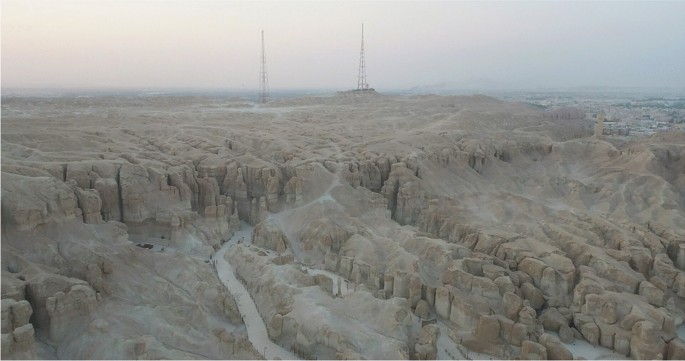The aerial photo captures a desolate, rocky bluff scene characterized by a dry, dusty, and desert-like landscape. The terrain is composed of jagged, brownish-gray rocks and boulders, split apart by deep crevices and cracks, giving an uneven and rugged appearance. A winding road snakes its way up the rocky mountain to a flat summit where two towering structures, likely radio or satellite towers, stand prominently. The overall ambiance is enhanced by a foggy, hazy sky, with dark white clouds lingering around the towers and the mountain's edges. In the distant background, to the top right of the image, there appears to be a small, indistinct town amidst some green patches, albeit blurry and difficult to discern with certainty. The starkness of the rocky cliffs and the contrasting metallic towers create a striking image of isolation and rugged beauty.